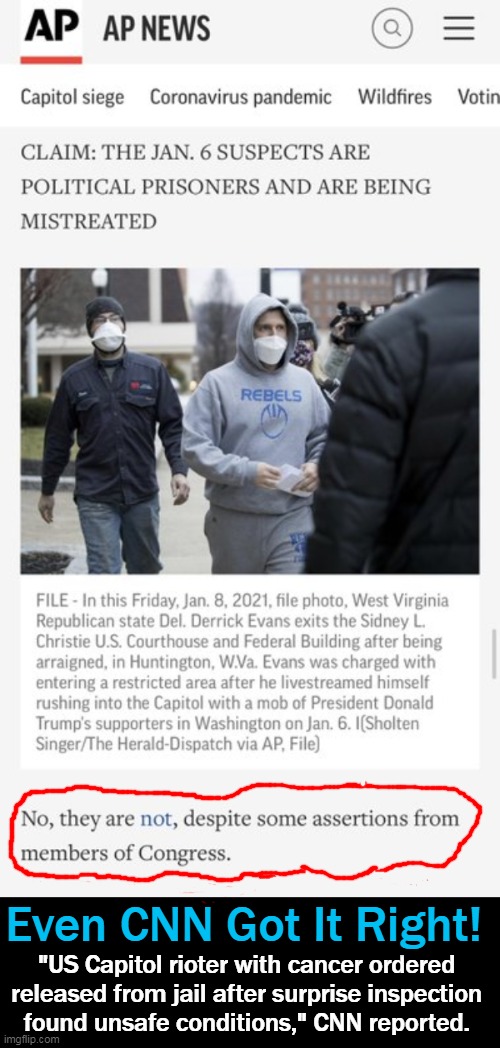This image shows a screenshot of an AP News article, likely taken from a mobile device. At the top, there is a grey header with "AP" in large text, followed by a search bar positioned on the right side and a menu icon represented by three horizontal lines. Below the header, there are clickable subjects in a white box with grey text: "Coronavirus," "Pandemic," "Wildfires," and a partially visible word that seems to be "Voting."

The main content starts with a grey text box featuring a controversial claim: "January 6 suspects are political prisoners and are being mistreated." Accompanying the text is a photograph of several men, presumably the January 6 suspects. The article's body text begins with a timestamp, "File in this Friday, January 8, 2021 file photo," and continues beyond what is visible in the image.

Towards the bottom, a specific segment is highlighted: "No, they are not, despite some assertions from members of Congress." Below this excerpt, there is a black text box containing additional information: "Even CNN got it right. U.S. Temple rioter with cancer ordered release from jail after surprise inspection found unsafe conditions, CNN reported."